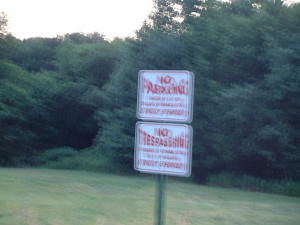This daytime photograph, though small and somewhat blurry, captures a no parking sign atop a no trespassing sign, both mounted on a green, weathered post. The signs feature prominent red lettering against a white background, with additional red text underneath that is illegible due to the image's graininess. The scene is set against a backdrop of patchy green grass and a dense, lush array of trees, with a faint orange glow in the sky just visible above the treeline. The photograph's simplicity and the limited visibility of its elements lend it a somewhat melancholic and mysterious atmosphere.